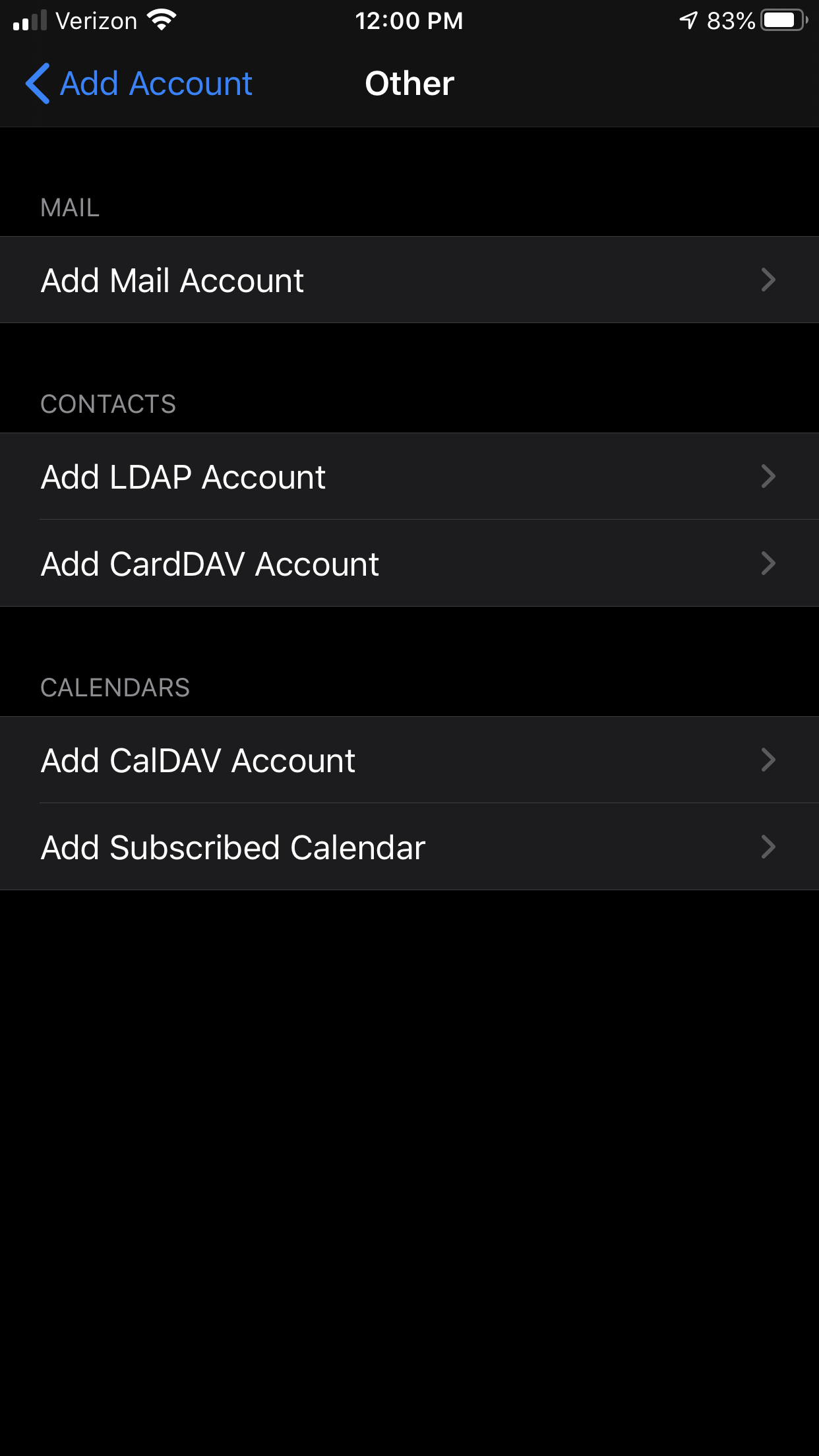The image depicts a smartphone screen with a predominantly black background. At the very top, the status bar displays several elements in white: signal strength bars, the text "Verizon," a Wi-Fi icon, the time "12:00 PM," and the battery level at 83%. Below the status bar, a blue section features a left-facing arrow next to the text "Add Account." Directly beneath this, the word "Other" appears in white.

Further down, the screen content flows in a structured manner. The label "MAIL" is presented in lighter gray and in all capitals. Underneath it, there's a box where you can add a mail account, indicated by a right-facing arrow. Following this, the label "CONTACTS," also in lighter gray and capital letters, appears. The options "Add LDAP Account" and "Add CardDAV Account" are listed below, each accompanied by a right-facing arrow.

At the bottom of the image, the label "CALENDARS," again in lighter gray and in capital letters, is followed by two options: "Add CalDAV Account" and "Add Subscribed Calendar." The latter follows a title case format while "Add CalDAV Account" uses a distinctive capitalization style ("CalDAV"), with the forward arrows pointing right next to each option.